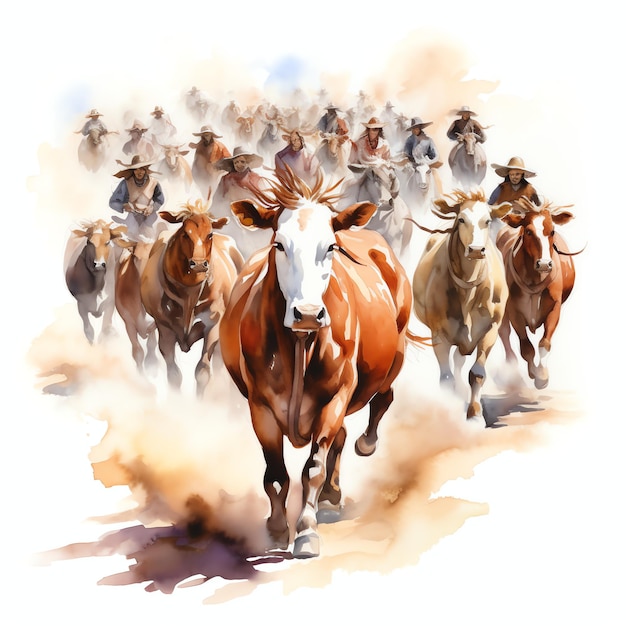The image is a graphic painting set against a white background that vividly portrays a dynamic herd of cattle being driven towards the viewer. At the forefront, a large brown and white cow with a white face and tufts of hair in the air appears to be galloping with one back leg raised, creating a sense of motion and urgency. Dust billows beneath its hooves, blending into the abstract watercolor-like depiction of the ground, which features swirls of dark brown, light brown, amber, and gold. Surrounding the lead cow, other cattle of varying shades of brown and beige are also charging forward, with two cows on the right and three on the left in the mid-distance. In the background, though faint and less defined, numerous figures of men on horses can be observed, likely about twenty, all wearing wide-brimmed hats, vests, and long sleeve shirts, reinforcing the scene of a classic cattle drive.